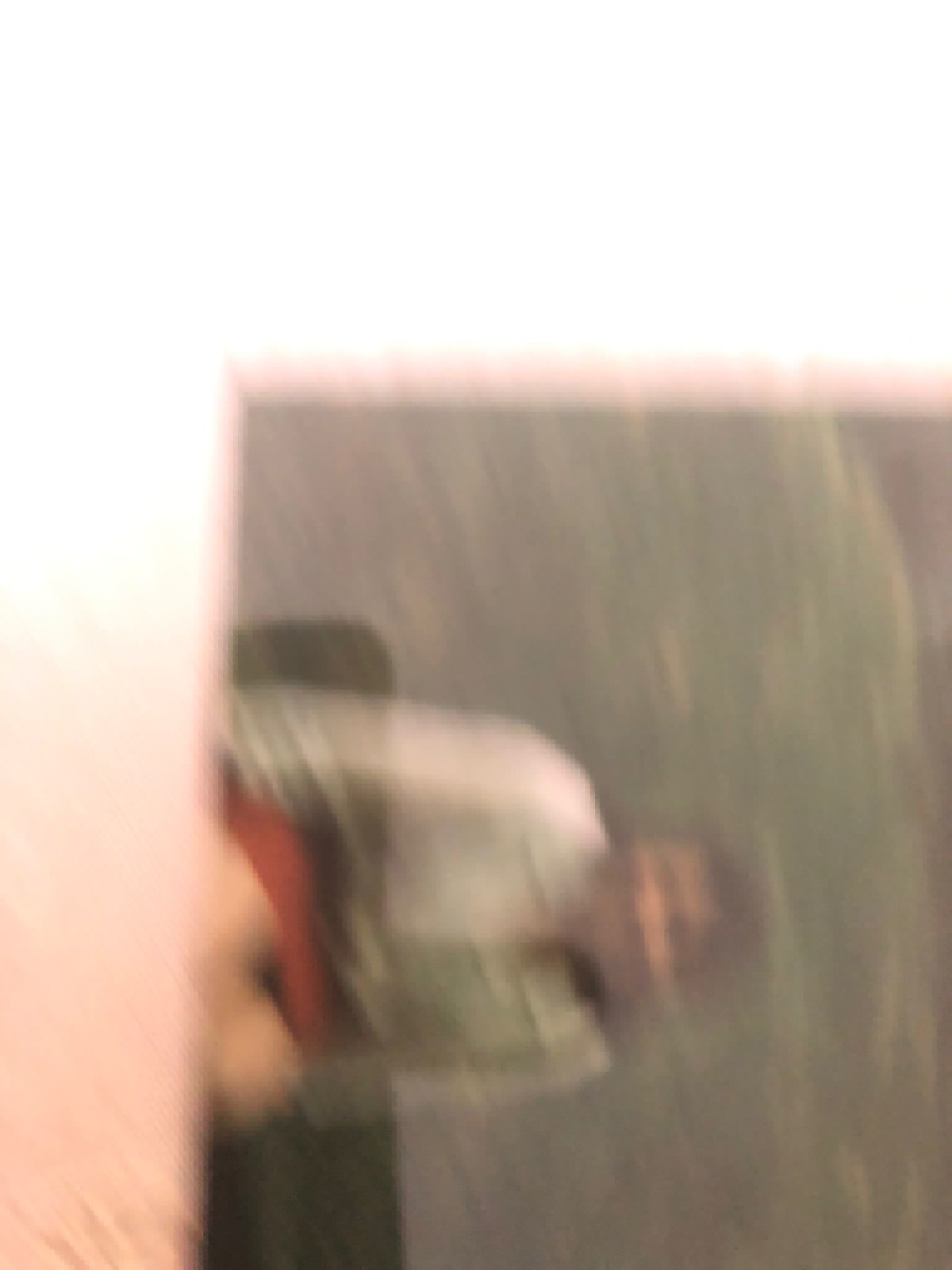This color photograph is significantly blurred and seemingly rotated to the right, making it visually challenging to interpret. The scene features a person sitting on a black couch, with their head pointing toward the right and their body toward the left. The individual is dressed in a white top and a red skirt or red shorts, with their knees exposed. Details of the person's features and background elements are indistinct due to the blurriness and possible multiple exposures.

The backdrop of the image is predominantly light-colored, transitioning from white at the top and left to a peachy or pale yellow-orange toward the bottom. Additionally, there is a notable grey wall behind the person, with a grey shadow seemingly passing through them. The black wall behind the individual has pink borders, and a pink object is visible in the bottom left corner of the image. Surrounding the main figure, who appears to have their hand resting on their thigh, there is a lot of greenery in the background, suggesting an outdoor setting with muted tones throughout the scene.